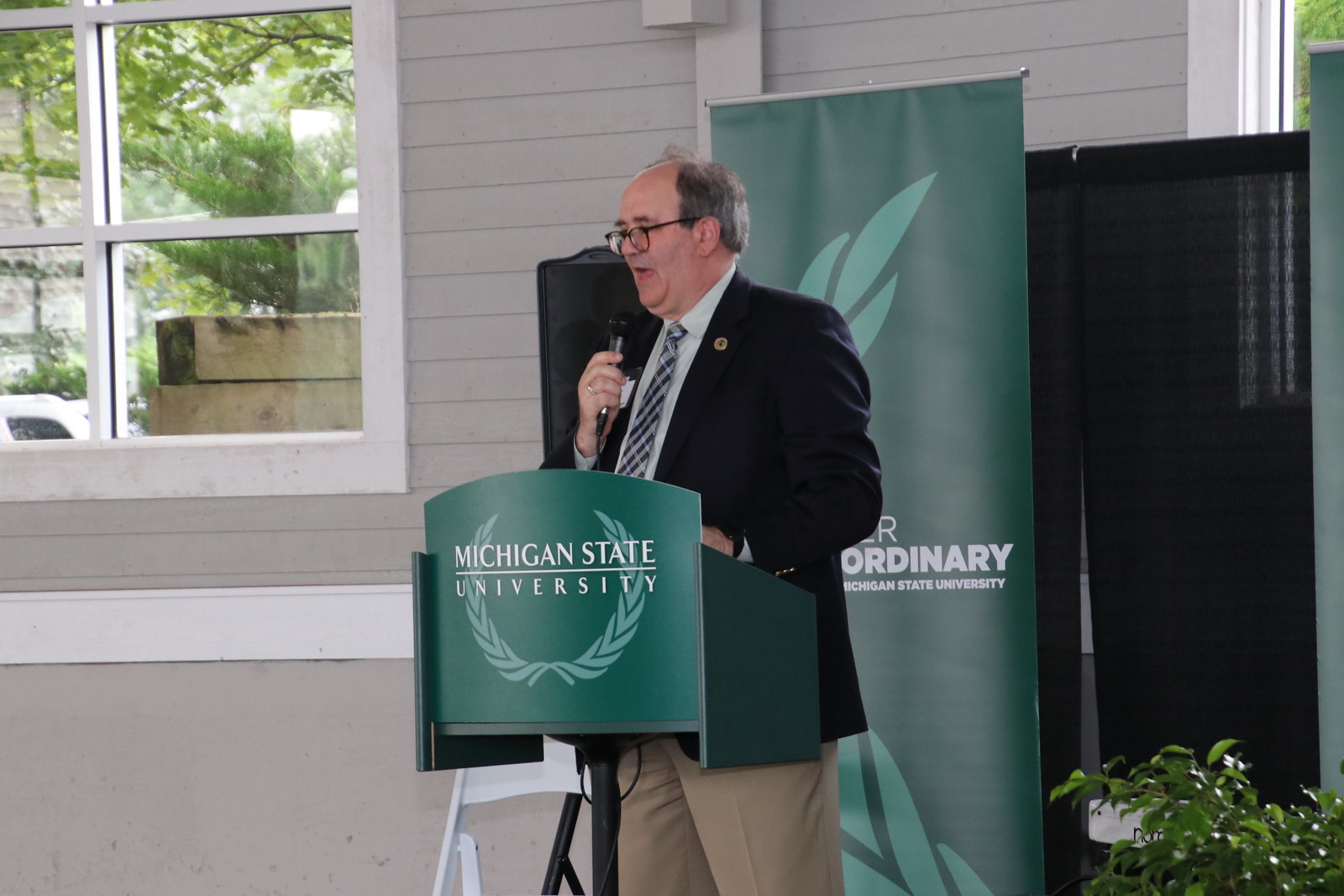In this color photograph, the primary subject is a man in his 50s or 60s standing at a podium outside a gray building with gray siding and white window frames. The surroundings reflect a bright, sunny day. The man, who has a receding hairline with some gray hair and wears round black glasses, is speaking into a microphone held in his right hand. He is dressed in a blue suit jacket, a white shirt, a blue striped tie, and tan khaki pants. The dark green podium features a wheat symbol and the words "Michigan State University" are printed on it. Behind the man is a vertical poster displaying a partially visible light green wreath and cut-off white text also related to Michigan State University. The backdrop includes a black curtain and some trees, as well as small bushes in front. Reflections of trees are visible in the glass window behind him, adding to the outdoor ambiance of the event.